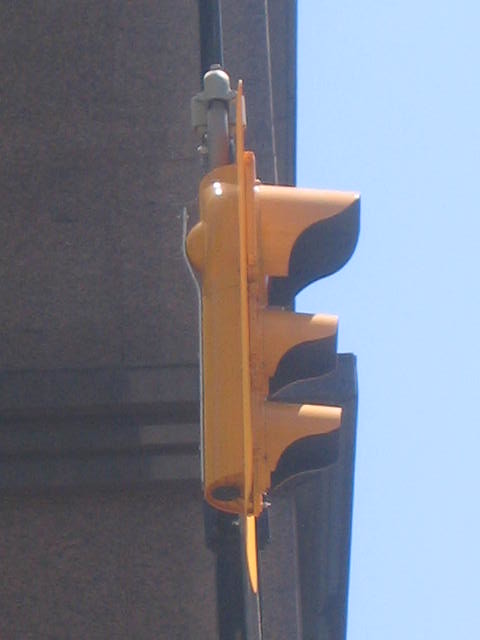This color photograph, taken in portrait format, showcases a close-up of a heavy-duty, yellow-painted traffic light from the side. The light is mounted on a black pole and appears sturdier and bulkier than usual, possibly due to it being an older model or designed to withstand harsh conditions. Captured from a lower, diagonal upward angle, the image prominently displays the traffic light as the main subject. Despite not revealing the red, amber, and green lights due to the side perspective, the robust yellow housing is evident. The backdrop features a concrete high-rise building without visible windows on the left and a clear blue sky on the right, emphasizing the urban setting and the distinctive traffic light.